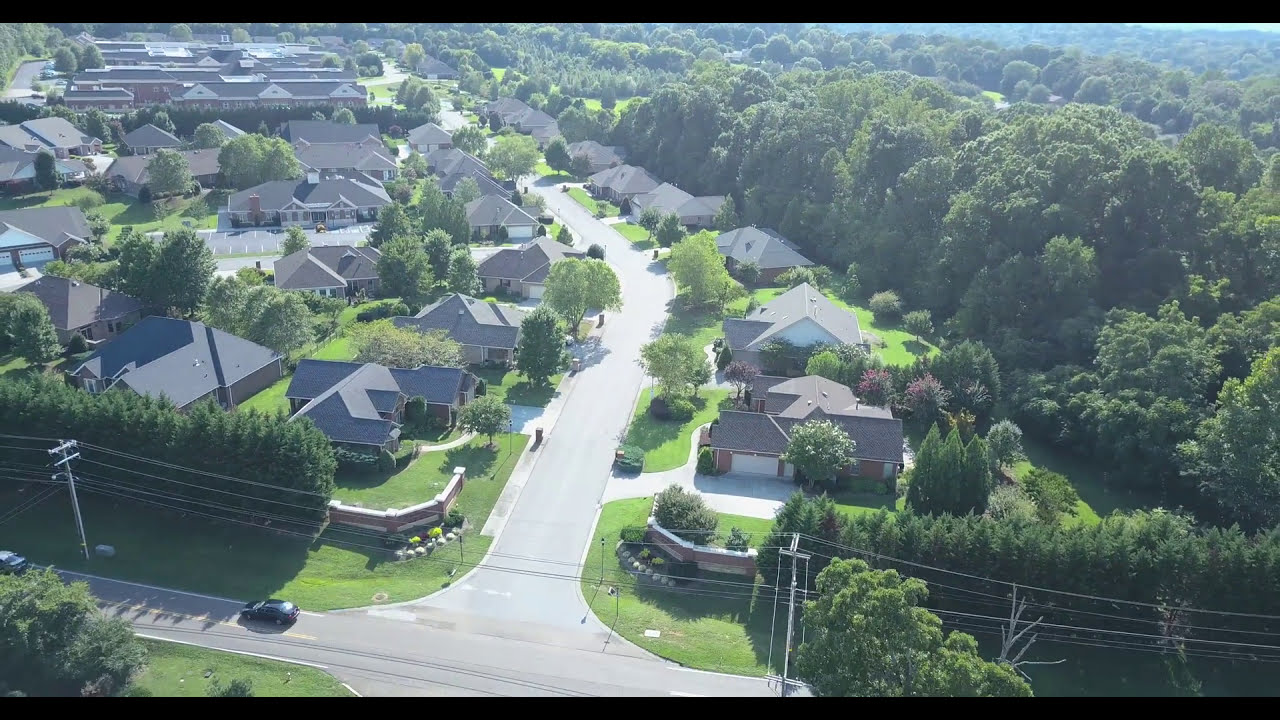This aerial photo depicts a serene, newer residential suburban area characterized by a main road that winds through rows of bungalow-style homes. The rooftops of these homes are predominantly dark gray with pointed, triangular shapes, and some feature white garage doors. The lush greenery is a prominent feature, with dense, massive trees creating a natural barrier around the neighborhood, ensuring privacy and an abundance of shade.

The vibrant, green lawns indicate a well-maintained community, likely captured on a sunny summer day, as suggested by the bright lighting. The main road cutting through the center of the image runs vertically before curving to the left and intersects with a horizontal road near the bottom of the photo. Along these roads, telephone poles and wires are visible, with two cars driving along the main thoroughfare, while some houses have garbage cans out for collection.

In the distant left-hand side of the image, the landscape transitions from residential homes to long, low rectangular buildings that may be commercial properties. The overall scene conveys a typical suburban setting with a harmonious blend of nature and carefully planned housing.